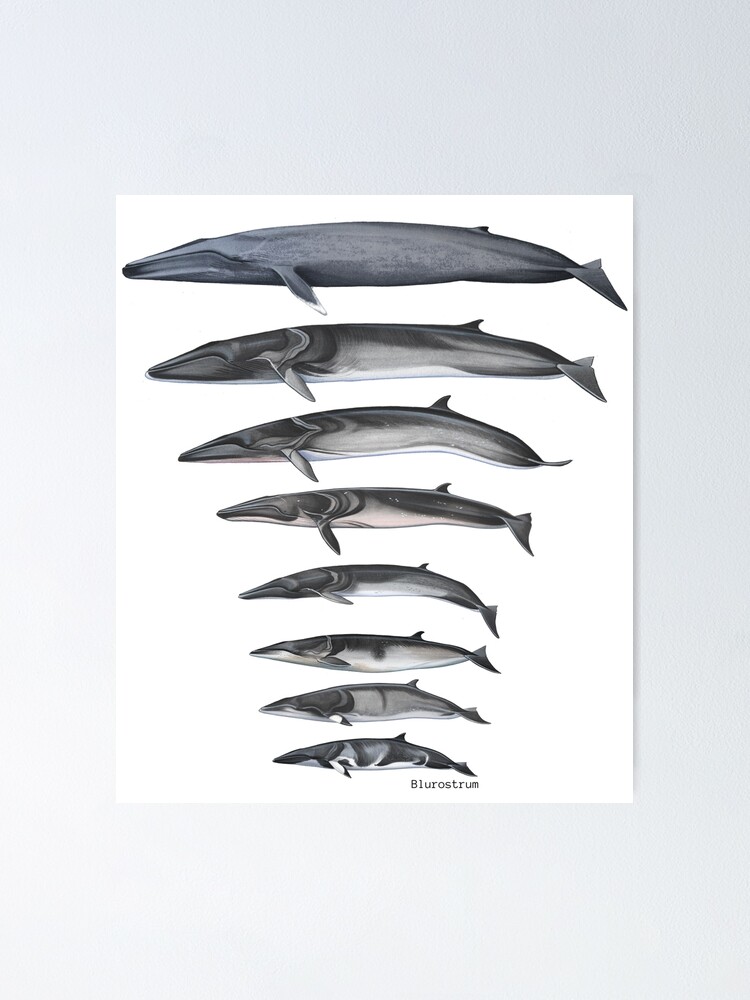The image features a detailed product photo of a poster displayed on a blank white wall. This poster illustrates eight different whales, arranging them from the largest at the top to the smallest at the bottom. The depicted whales range in size, with the smallest being approximately a third to a fourth of the size of the largest. Each whale is predominantly gray, with the one at the top exhibiting a bluish tint, suggesting it might be a blue whale. The coloration fades to darker shades of gray as you progress down the poster. The background of the poster is white, creating a stark contrast with each whale's silhouette. The only text present on the poster is a watermark or brand name, "Blue Rostrum," positioned at the bottom.